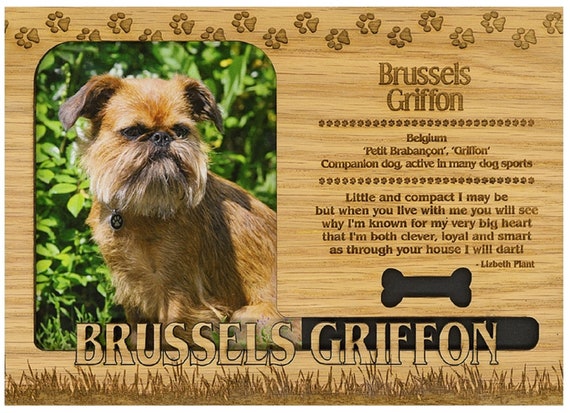The image depicts a detailed placard featuring a Brussels Griffon dog with a scruffy, tan to brown coat and a characteristic squished face, accentuated by strong grayish-brown facial hair. The dog, medium to small in size, wears a collar adorned with a small paw print charm. The central picture of the dog is placed within a rounded-edge rectangular frame, set against a green grassy area with foliage in the background. The placard has a distinctly distressed, light brown wooden or paper-themed border, with small paw prints at the top and brown animated grass at the bottom. Underneath the dog's image, the words "Brussels Griffon" are prominently displayed, followed by descriptive text that reads: "Belgium Petit Barbet Griffon – companion dog, active in many dog sports. Little and compact I may be, but when you live with me, you will see why I'm known for my very big heart. I’m both clever, loyal, and smart. As through your house, I will dart." The attribution "By Lisbeth Plant" is noted near the bottom, along with a small black graphic of a dog bone.